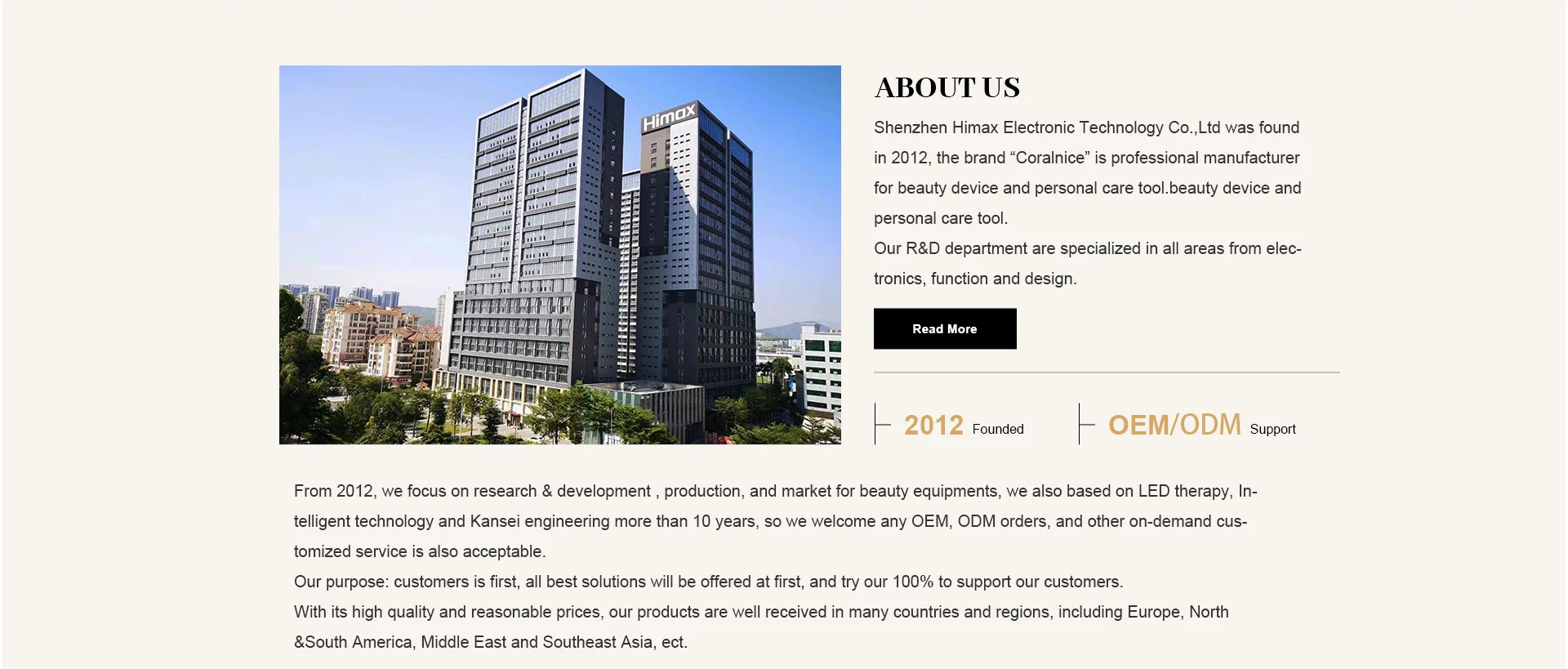**Screenshot of a Technology Company’s “About Us” Page**

The screenshot appears to be from the “About Us” page of a technology company’s website. In the upper left corner, there is a photograph of a tall building, likely situated in a city. The structure of the building is unique, with multiple sections creating a near-square shape.

To the right of the photograph, bold capital letters spell out “ABOUT US.” Below this heading, text states, "Cheyenne Hymax Electronic Technology Company Limited was founded in 2012. The brand Coral Nice is a professional manufacturer of beauty devices and personal care tools." This phrase, "beauty device and personal care tool," is repeated twice.

Further down, a brief description highlights the company's Research and Development department, which specializes in electronics, functionality, and design. There is a black button labeled "Read More."

Underneath this section, important details are displayed: "2012 founded" and "OEM/ODM support," both in a faded dark orange color.

Following this, a couple of paragraphs elaborate on the company’s focus since its inception in 2012. The text explains their commitment to research, development, production, and marketing of beauty equipment, particularly leveraging LED therapy, intelligent technology, and Kansi engineering. It also emphasizes their readiness to accommodate OEM and ODM orders and other customized services on demand.